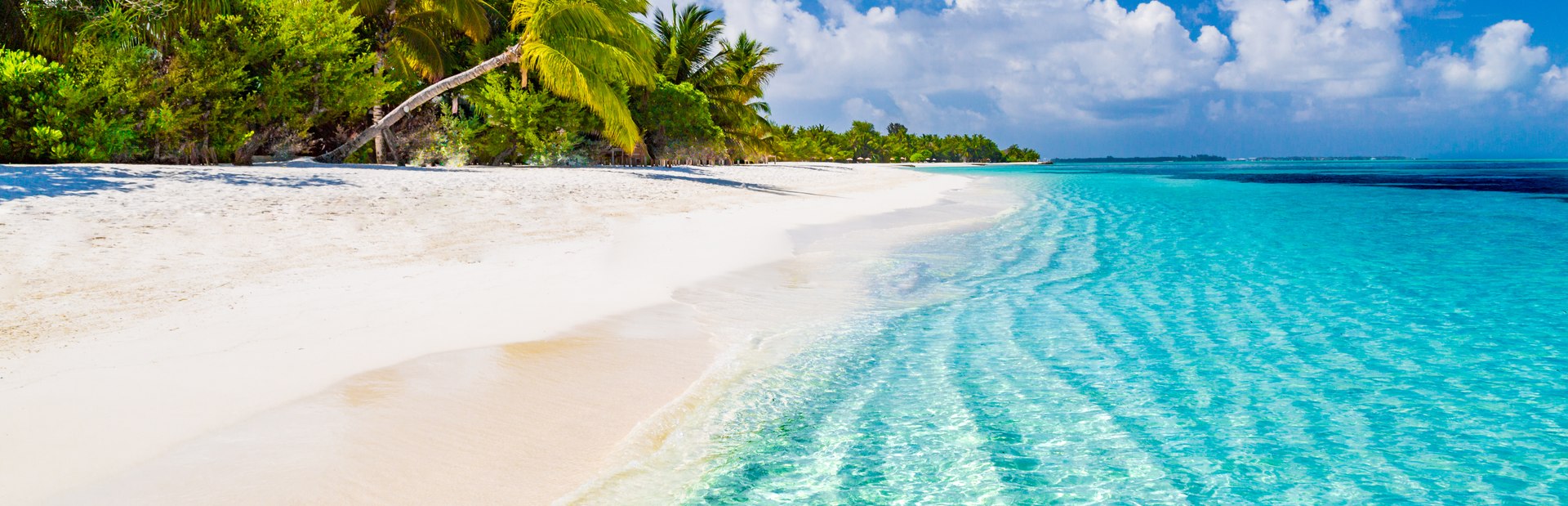This photograph captures the serene beauty of a tropical beach, evocative of the Caribbean. On the right-hand side, the crystal clear, aqua-blue waters gently lap against the pale sand of the beach, revealing the ocean floor beneath. The water is calm, with only small, gentle waves. In the far distance on the right, a small peninsula dotted with trees juts out into the ocean. The sky above is a mix of blue and bright white clouds, suggesting a sunny day, although there are hints of possible rain far off in the background. 

On the left-hand side, the beach extends further than the eye can see, bordered by lush, vibrant greenery. The upper left corner features tall, healthy palm trees and dense shrubbery, contributing to the tropical ambiance. This stretch of land, dense with vegetation and featuring a wide variety of plant life, gives the impression of a large, verdant island. Overall, the image radiates an idyllic, tranquil atmosphere, embodying the essence of a perfect beach day.